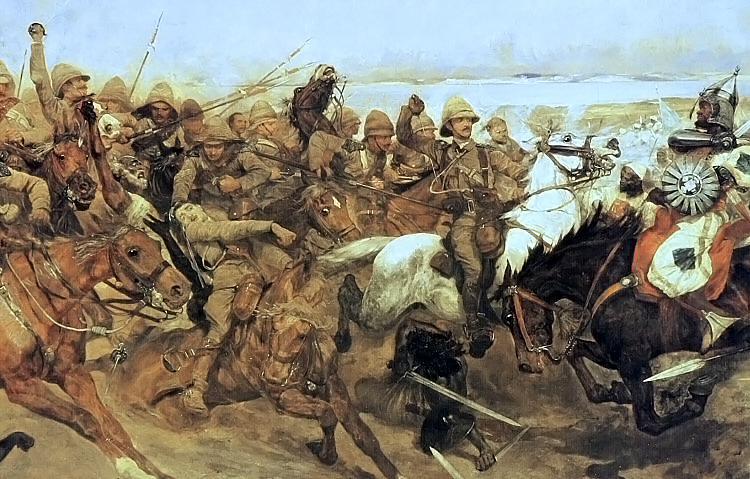This is a detailed painting depicting a chaotic war scene from a historical battle. The scene shows cavalrymen, possibly colonial soldiers, charging at another group that appears to have Medieval knight-like armor. The left side features men in explorer-like gear on brown horses, wearing golden yellowish green outfits. On the right side, men dressed in silver chain mail are riding black horses, indicating a more knightly appearance. Both sides are armed with a mix of swords, shields, spears, and guns.

The ground in the painting has a brownish hue, and the sky above is a somber gray, adding to the neutral and tense atmosphere. The clothing and armor colors vary from tan, beige, and white to darker tones like black and dark gray. The chaotic composition shows men falling off horses, weapons raised, and expressions of terror and anger on their faces. Horses are depicted mid-rear, with open mouths, adding to the sense of frantic motion and high stakes of the battle. This painting captures a moment of intense conflict and struggle, with detail in both attire and emotion.